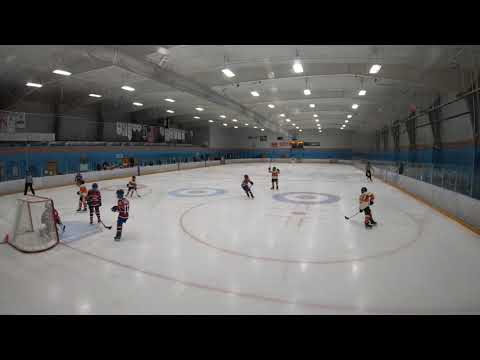The image portrays an indoor ice hockey rink where a team of mostly young players, possibly around ten years old, is practicing. The rink's white ice surface is marked with red lines and blue circles specific to hockey play. Surrounding the rink is a fence with a white top and yellow bottom, and the walls of the facility are painted white on the upper portion, with blue on the lower part and a yellow stripe in between. There are eight to nine children on the ice along with a coach. The players are wearing jerseys that are either red with white accents or white with red accents. The scene also includes a goalie positioned near a goal with a red rim and white net, appearing to either defend or return a shot. The ceiling is white with visible support beams and installed lights, illuminating the large indoor space.